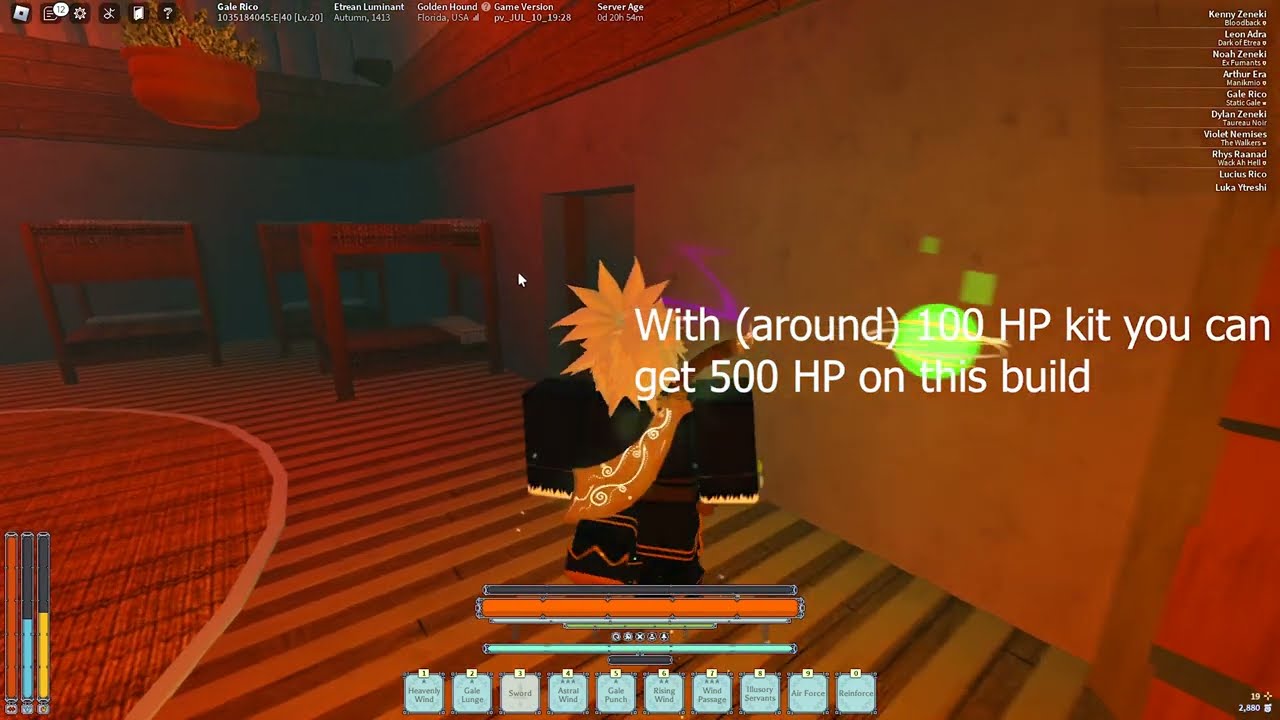The image is a computer-generated screenshot from the Roblox video game, depicting a dimly lit room bathed in red light. The room has cement walls and a floor made of alternating light and dark wood, partially covered by a round, graph-patterned rug. In the upper left corner, three wooden bunk beds are arranged. Notably, a character with spiky orange hair, dressed in a black suit with orange and white accents, stands in the central foreground. Above the character, an orange health bar is visible, and nearby in white text, it reads, "With around 100 HP kit you can get 500 HP on this build." The bottom of the image features orange, blue, and red bars next to a series of small square icons, while the upper corners contain small black icons with white graphics and unreadable white text likely showing player names and other data. Additionally, a doorway is visible near the beds, and a plant hangs from the ceiling.